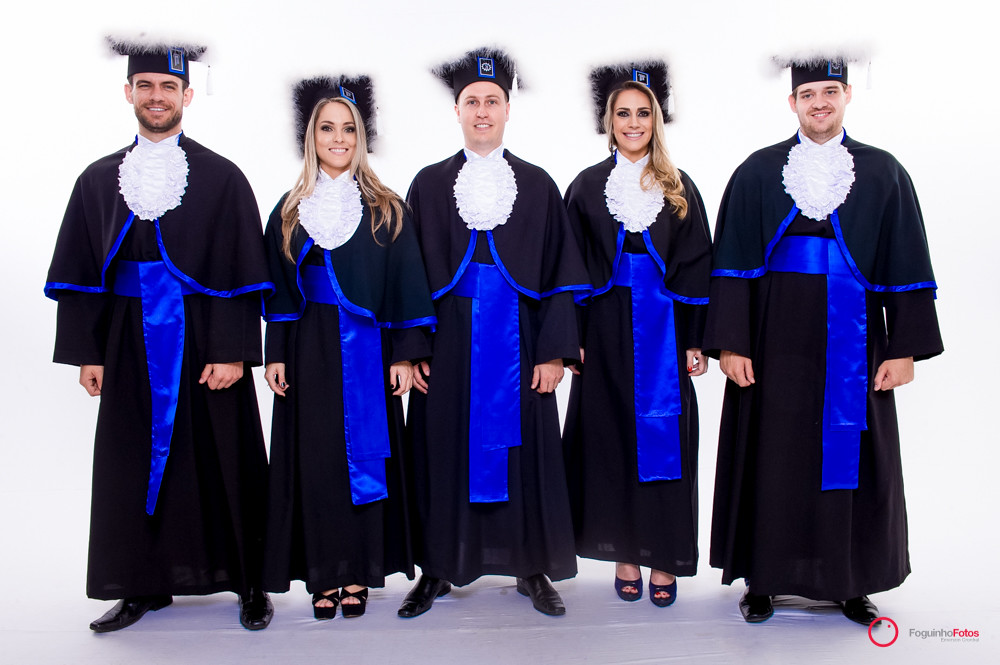The photograph features five Caucasian individuals—two women and three men—standing shoulder to shoulder in a neat row. From left to right, the order is a man, a woman, a man, a woman, and a man. Each person is adorned in a black robe elegantly trimmed with royal blue, complete with a blue sash around the waist. Their costumes include a distinctive frilly white collar that adds a formal touch to their attire. The men have short black hair, with one sporting a beard and mustache while the other two are clean-shaven. The women, who have long blonde hair, bear a striking resemblance to each other, almost suggesting they could be sisters. Atop their heads are black hats resembling graduation caps, but unique in that the tops are adorned with fluffy white material. The background is uniformly white, and the floor they stand on is also white, creating a clean and minimalist setting. In the lower right-hand corner of the image, the text "Foginho Photos" is displayed in red lettering. The top parts of their hats merge into a cloudy and fuzzy effect, further emphasizing the surreal quality of the altered photograph.